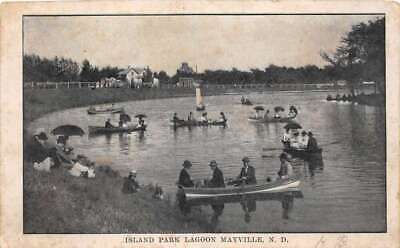This black and white photograph, which appears weathered and slightly yellowed with age, captures a vintage scene on what is labeled at the bottom as Island Park Lagoon, Mayville, MD (or possibly North Dakota). The image shows a serene lake or pond surrounded by a curved shoreline. In the water, there are about seven long, narrow canoes, each occupied by three to four people—both men and women. The men are dressed in suit jackets with hats, while the women wear long dresses and hold umbrella shades for protection from the sun.

To the left of the lake, several people, likely spectators, sit on a grassy area observing the boaters. The atmosphere conveyed is one of leisure and community gathering. In the background, beyond a fence, a white house is visible, along with a row of trees, adding depth to the scene. The sky overhead is clear, enhancing the timeless quality of the photograph.